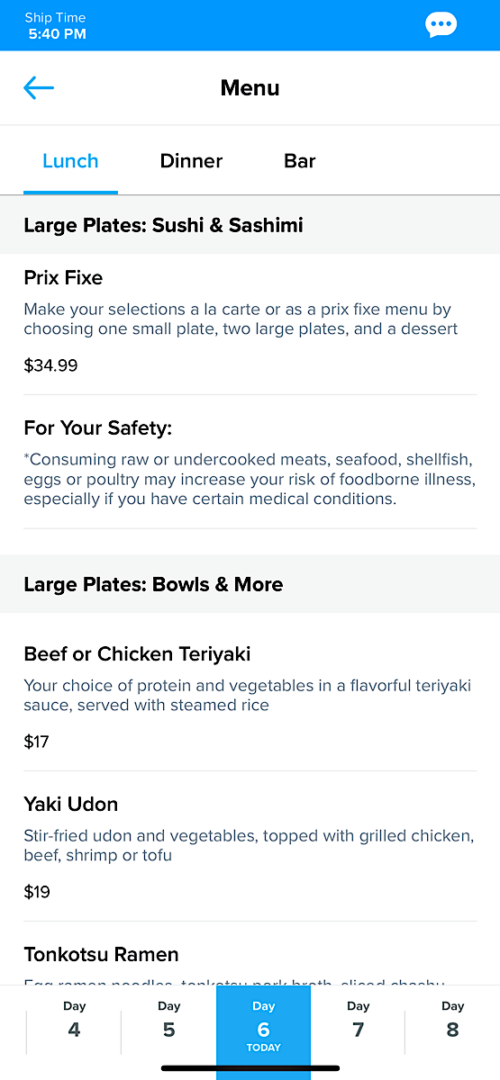This screenshot captures the interface of a mobile application featuring the menu of an Asian restaurant. At the top, it displays the word "Menu" with a blue left-facing arrow to its left. Below that, there are selectable options for different meal times: "Lunch," "Dinner," and "Bar." The "Lunch" menu is currently in focus, indicated by its blue highlight, while "Dinner" and "Bar" options are in black text.

The lunch menu is divided into several sections. The first section is titled "Large Plates: Sushi and Sashimi." Under this section, one item is listed: "Prix Fixe."

The next section is "Large Plates: Bowls and More," featuring multiple items including "Beef or Chicken Teriyaki," "Yaki Udon," and "Tonkotsu Ramen."

At the bottom of the screen, there is a horizontal strip displaying days of the week labeled "Day 4," "Day 5," "Day 6," "Day 7," and "Day 8." Currently, "Day 6" is highlighted in blue.

This detailed layout of the mobile application's menu provides a clear and organized view of the available meal options for lunch, segmented into specific categories for easy navigation.